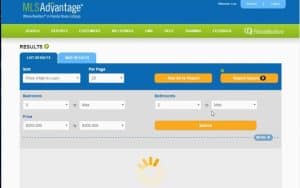The image depicts a very blurry webpage, likely related to healthcare. The top of the page features a blue bar with "MLS" in green lettering on the upper-left corner, accompanied by the word "Advantage" in white font. This suggests it is a medical website, although the low resolution makes it difficult to discern specific details. Below the blue bar, there is a green bar with several website options, though their exact labels are unclear. 

Prominently, at the top of the content area, there is a "Results" section in white text. A further green bar appears to contain additional options, including a black "Results" label adjacent to a green check mark. Below this, there are two tabs: the first being green and including a couple of yellow buttons, and the second being gray with what seems to be another button. At the bottom of the screen, a partial loading circle is visible. Despite the poor resolution of the image, the website's layout and color scheme are indicative of a standard local healthcare portal.